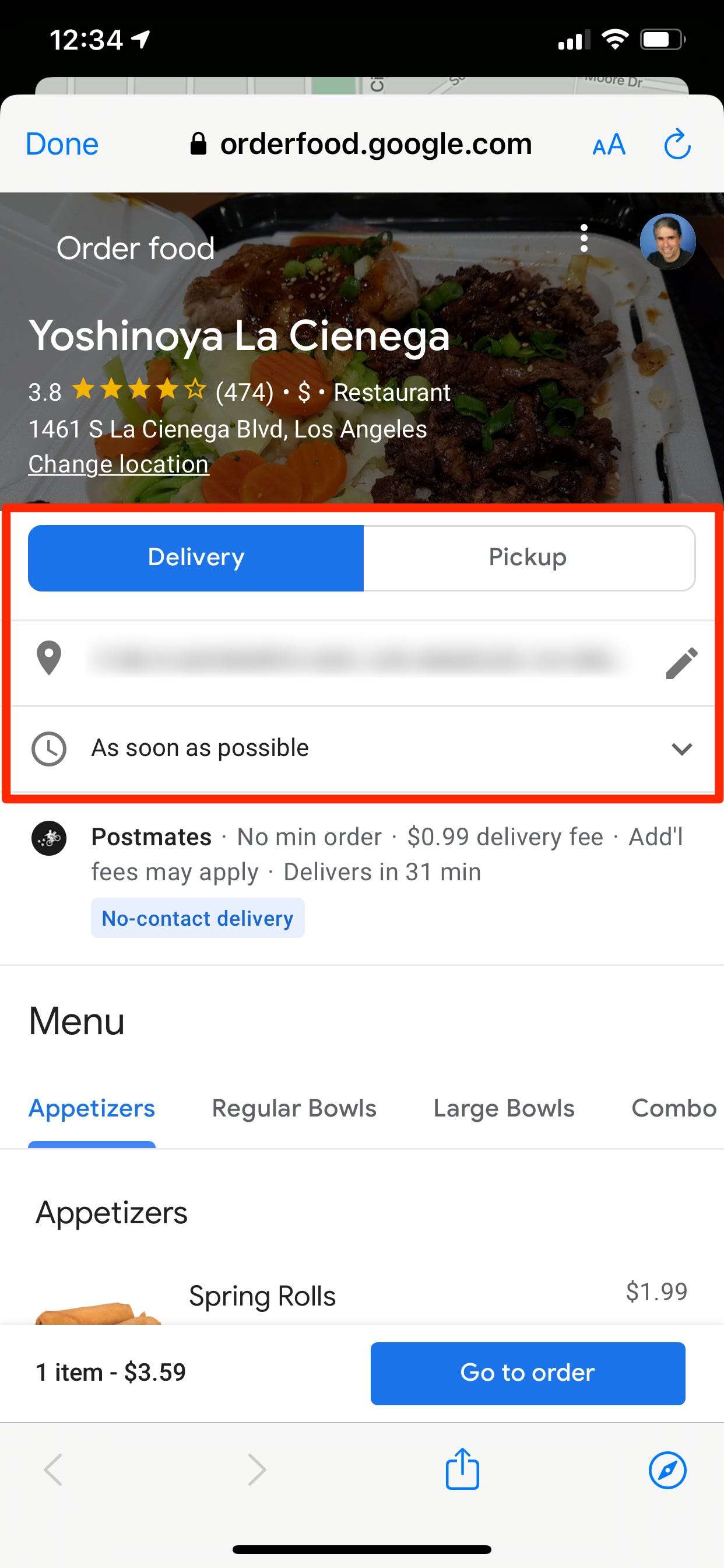A user is seen navigating orderfood.google.com on their smartphone, placing an order from Yoshinoya La Cienega. The restaurant, which boasts a rating of 3.8 stars from 474 reviews, is marked as budget-friendly with a single dollar sign ($) and is situated at 1461 S. La Cienega Boulevard, Los Angeles. 

A red box highlights the order options, allowing the user to choose between delivery and pickup. The map icon confirms the location, and the user has opted for the earliest available delivery. The details mention Postmates as the delivery service, with no minimum order requirement, a $0.99 delivery fee, potential additional fees, and an estimated delivery time of 31 minutes. A prominent blue button offers the choice of "no contact delivery."

Exploring the menu, appetizers are highlighted, featuring spring rolls for $1.99. Other menu categories available include regular bowls, large bowls, and combos. Currently, the user's cart contains one item priced at $3.59, with a "go to order" button ready for the final checkout process.